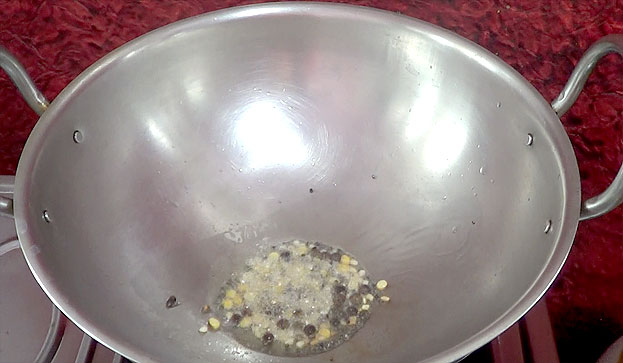A large silver strainer bowl dominates the center of the image, spanning close to the edges—about half an inch from the left and right sides. The bowl overlaps the bottom of the frame and touches the top. Reflections from two lights are visible on the upper part of the bowl, creating bright spots. Handles extend from both sides of the bowl, with the left handle reaching out of the frame.

Inside the strainer, there is a mix of water with yellow, black, and white particles, possibly some form of seasoning. The background features textures and colors that add depth to the image. On the left side, approximately halfway down the frame, there seems to be a backdrop resembling red shag carpet, which extends to about an inch from the bottom on the right side. 

Interspersed within this red background, on the left, a silver object that could be part of a stove is visible. It appears to come down and slightly underneath the bowl. On the right side of the bowl, there is a black space followed by two long red wooden pieces extending vertically under the bowl, separated by a thin black gap. The bottom right corner is predominantly black, except for a small intrusion of red fabric.

This intricate setup blends metallic tones with vibrant reds, creating a visually engaging scene centered around the well-used kitchen strainer.